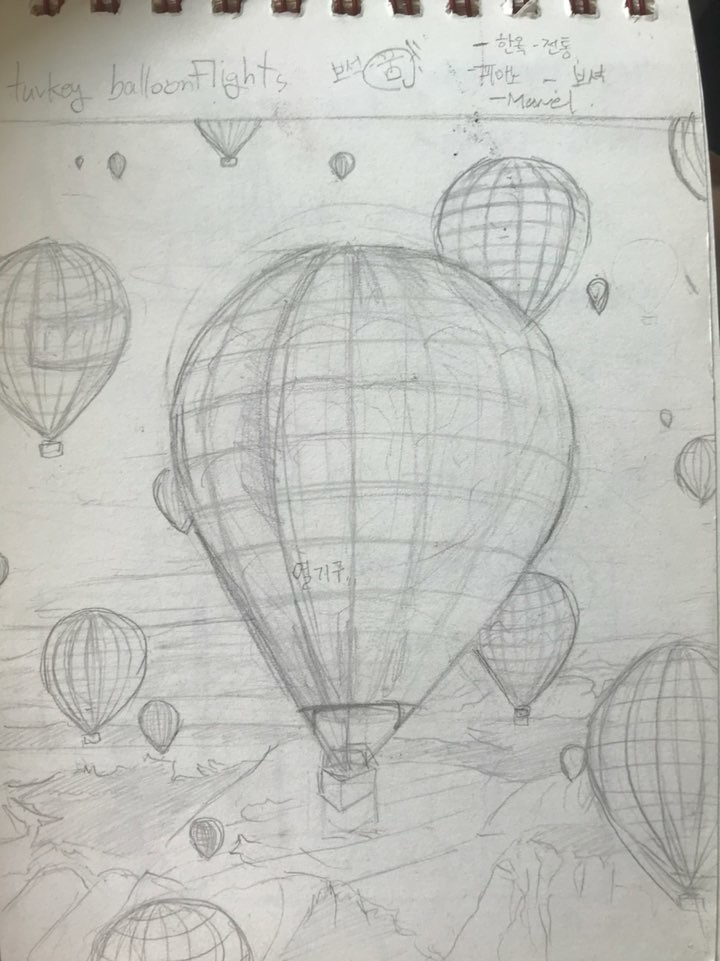This rectangular, vertically-oriented pencil sketch captures the enchanting experience of hot air balloon flights in Turkey. It appears to be drawn in a sketchbook, evidenced by the visible binding at the top. The top of the sketch features the words "Turkey Balloon Flights" in clear pencil print, and to the right, partially written in an unrecognized Asian script, there is a hint of the word "Marvel." Below this header, the artist has masterfully depicted a sky crowded with air balloons.

Dominating the foreground, and occupying nearly half the drawing, is a large, intricately shaded hot air balloon. The shading is subtly executed with vertical and horizontal pencil strokes, giving the balloon a textured appearance. The basket beneath the balloon is drawn three-dimensionally, though it’s unclear whether it contains people or merely shadows.

Surrounding this central balloon are six smaller balloons – three on the lower right and three on the left. At the sketch’s bottom left corner, the upper part of another balloon is visible. The lower section of the sketch is filled with swirling lines, suggesting either clouds through which the balloons drift or abstract terrain formations below them. The entire scene is rendered in pencil, bringing a soft, ethereal quality to this picturesque representation of a balloon-filled sky.